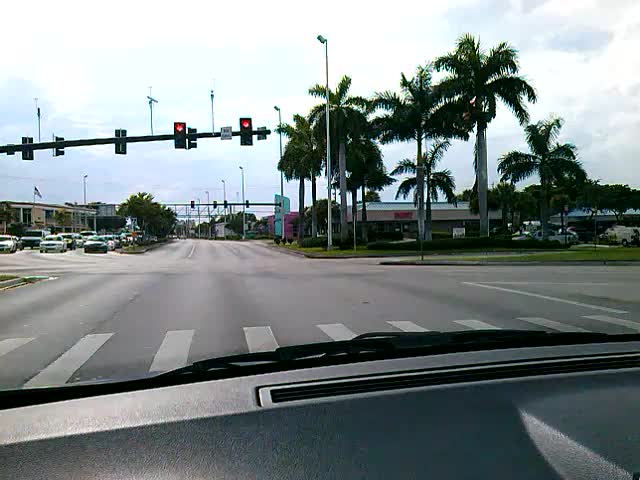This photograph captures the view from inside a car stopped at a red light, looking out through the front windshield onto a wide, multi-lane road. The car's medium-gray dashboard, with its window wipers, is partially visible in the foreground. Directly ahead, thick crosswalk lines stretch across the broad roadway. There are no cars in front of us, but across the street on the opposite side, several lanes are filled with cars stopped in the opposite direction.

To the right, there is a small shopping area with a lush green lawn dotted with beautiful palm trees. This area includes various buildings and parked cars, possibly suggesting a gas station or a bank. A yellow building with an American flag is also visible in the distance. Palm trees can be seen on the grass farther along the right side.

Above the road, in the upper left-hand corner, a traffic light hangs overhead, showing red. Scattered clouds fill the daytime sky, which appears mostly white with some gray. Additional streetlights line the road farther ahead, emphasizing the area’s broad, busy nature and hinting that it might be near a significant location such as an airport.